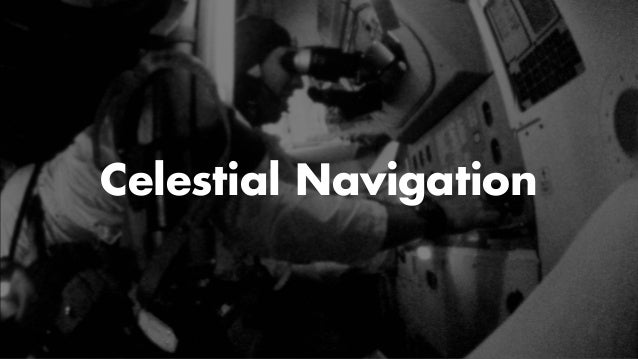In this black and white, slightly blurry photograph titled "Celestial Navigation," a man is shown meticulously operating intricate machinery within an enclosed, lab-like or possibly craft environment. He is looking intensely through a viewer or scope, appearing to make precise adjustments with his hands on various knobs or dials. The man is wearing long sleeves and a hat, with a scarf or helmet strap wrapped around his chin, emphasizing a sense of focus and preparation. Despite the lack of clear detail due to the photo’s blurriness, the scene conveys a meticulous operation possibly related to navigation, whether it be undersea, airborne, or astronomical, as suggested by the prominent white text reading "Celestial Navigation" at the center of the image.